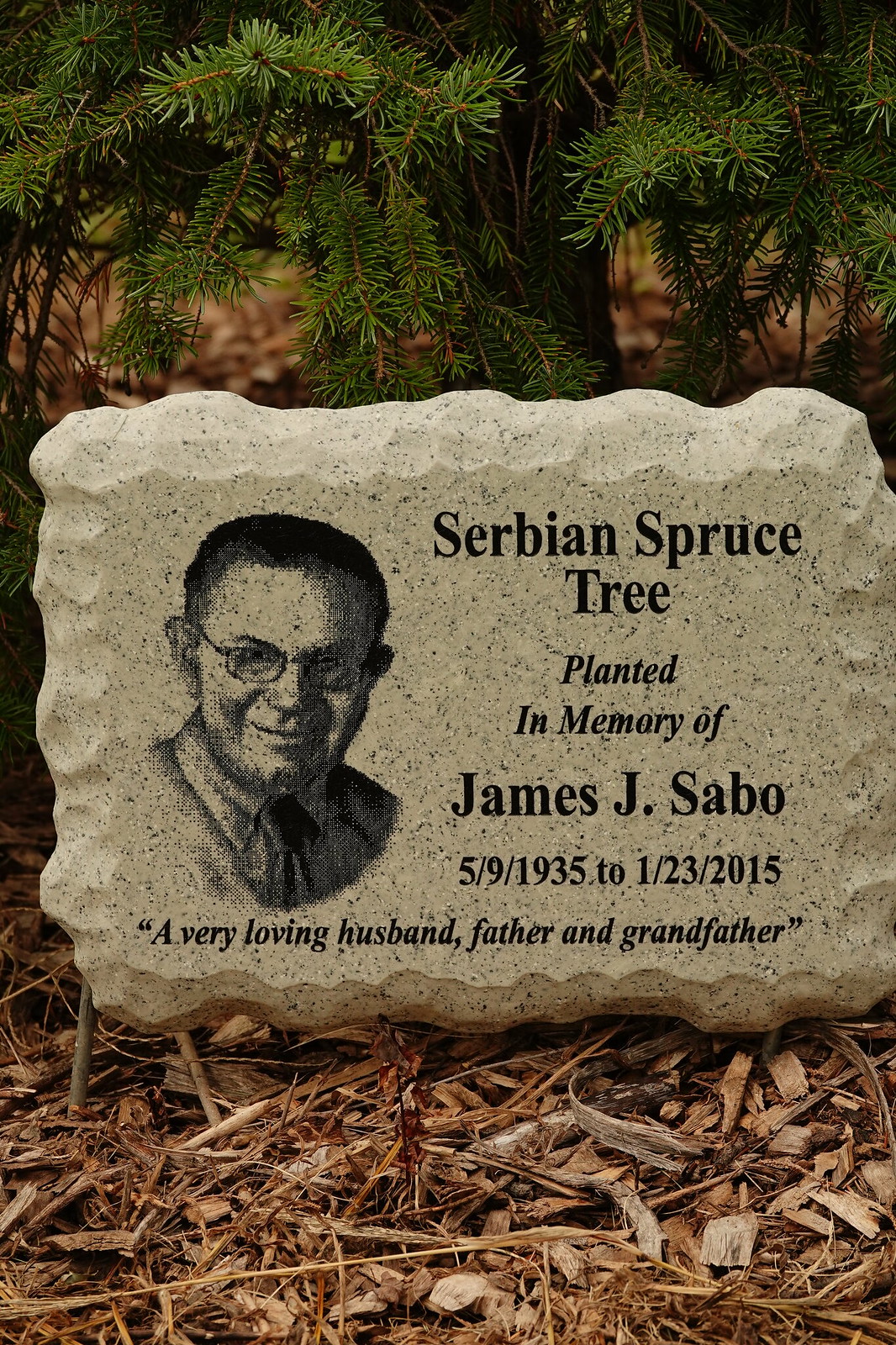The image shows an outdoor memorial set against a backdrop of blurred brown foliage and needles from an evergreen tree. 

In the foreground, there is a prominent man-made rectangular rock formation with rippled edges. The formation sits atop a bed of brown mulch and dead bark. A black-and-white photograph of a gentleman wearing glasses is printed on the rock, along with an inscription that reads: "Serbian spruce tree planted in memory of James J. Sabo, 5-9-1935 to 1-23-2015, a very loving husband, father, and grandfather."

Above the memorial, a Serbian spruce tree stands tall, honoring the memory of James J. Sabo. The entire scene is contained within a vertical rectangle, with the headstone centrally positioned amid the natural elements surrounding it.